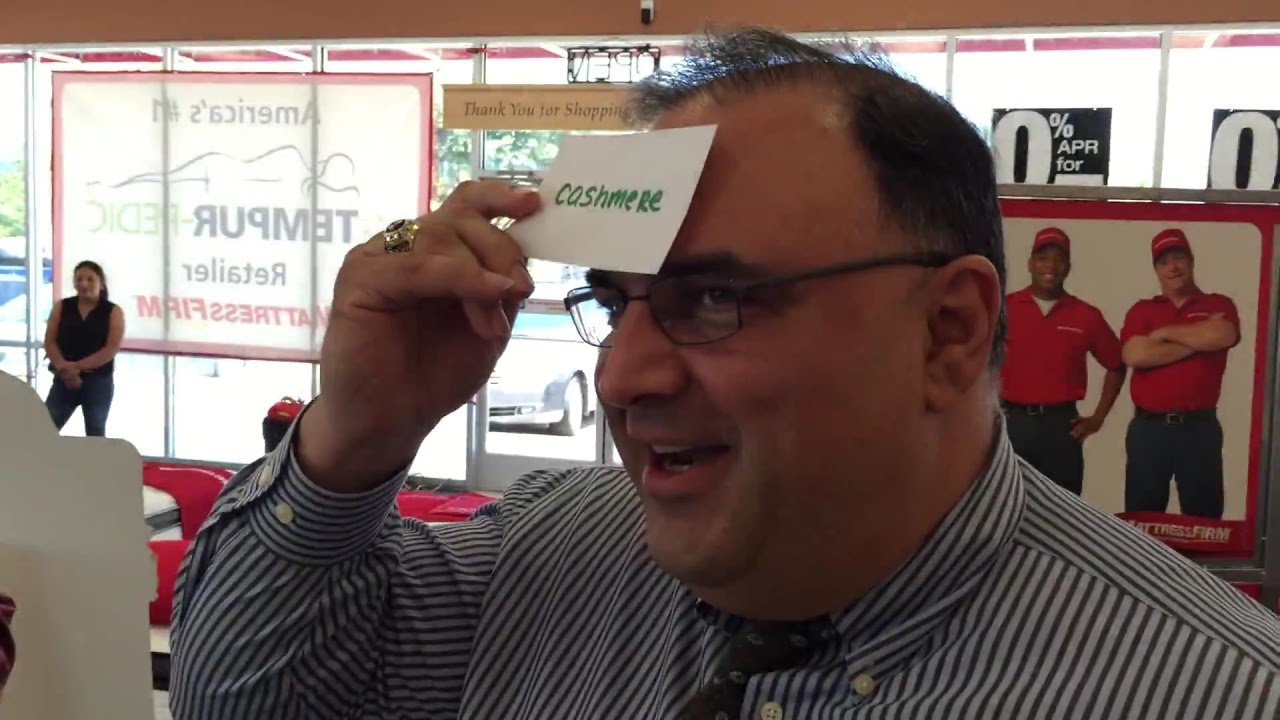The image depicts an older, slightly plump man with thinning black hair and thin black glasses, wearing a long-sleeve, button-down dress shirt with vertical dark blue or dark gray stripes on a white background. He has a blue tie and wears a large sovereign ring on the fourth finger of his right hand. The man is holding a white card with green letters spelling "cashmere" to his forehead, suggesting a game. He seems to be smiling with his mouth open and is facing slightly to the left. The setting appears to be a store, likely a Mattress Firm or Tempur-Pedic retailer, as indicated by the signage and posters visible in the background. Over his left shoulder is a glass window with a reversed sign reading "America's number one Tempur-Pedic retailer mattress firm." In the upper left corner of the image, a woman with a black sleeveless blouse and black pants is standing in front of a window. A poster featuring two men in red uniforms with red caps is also visible, partly obscuring a black sign with white lettering that hints at a car dealership or repair shop. The scene gives off a casual, somewhat playful atmosphere centered around the man engaging with the card game.